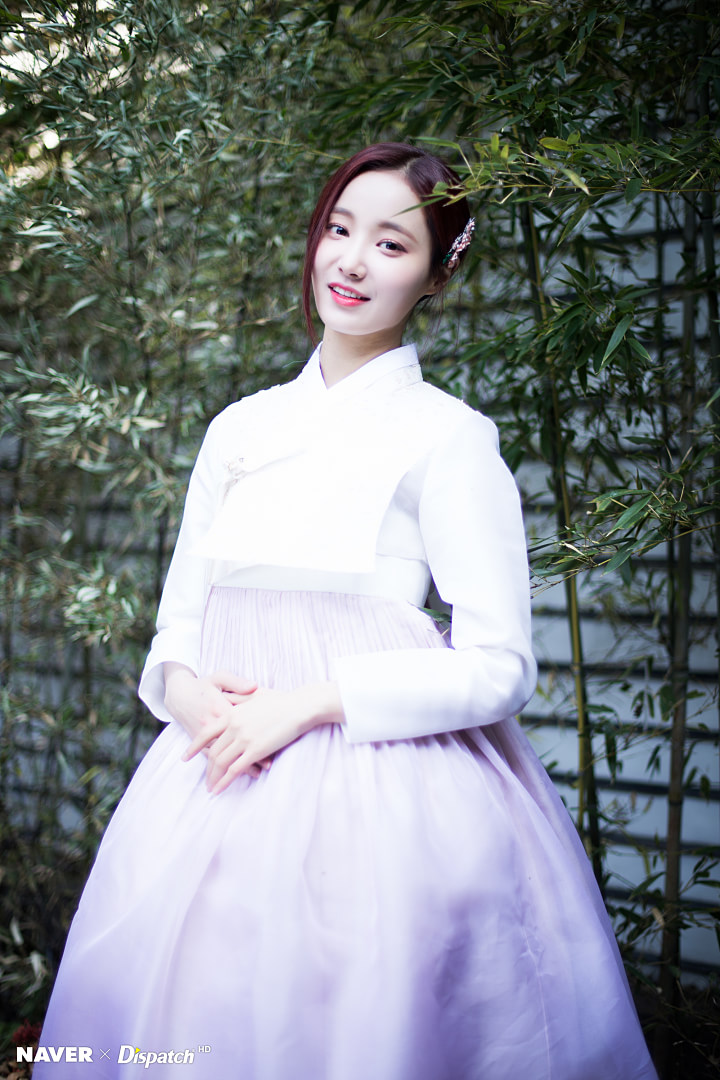The image depicts an Asian woman in front of a white wall with window blinds and bamboo plants. She is wearing a traditional-style dress, featuring a white top with a high collar and a loose, square chest part. Her full skirt is a very light purple or pink color and flares out dramatically, resembling a ball gown. The woman has dark brown hair, adorned with a hairpin or barrette on the right side, and her skin appears almost powder white due to a lighting effect in the photograph. Her brown eyes are complemented by bright red or pinkish lipstick, and her head is tilted slightly to the right with a soft smile. Her hands are delicately placed one over the other. In the bottom left corner, small white text reads "NAVER x DISPATCH HD."